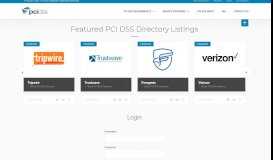A small and somewhat blurry screenshot of a website for a company possibly named "PCI.SS" is displayed. The layout features a white background with the company’s blue logo positioned in the upper left-hand corner. To the right of the logo, stretching from the middle to the top right of the image, are five distinct links or pull-down menus providing navigation to various parts of the website.

Beneath the menu bar, a bold heading reads “Featured PCI OSS Directory Listings.” Underneath this heading, four images are arranged horizontally. The first image on the left is linked to Tripwire, while the second image displays an indistinguishable company logo. The third image features an unidentifiable logo, and the fourth image links to Verizon.

At the bottom of the screenshot is a login section where users can enter their username and password to access their accounts.